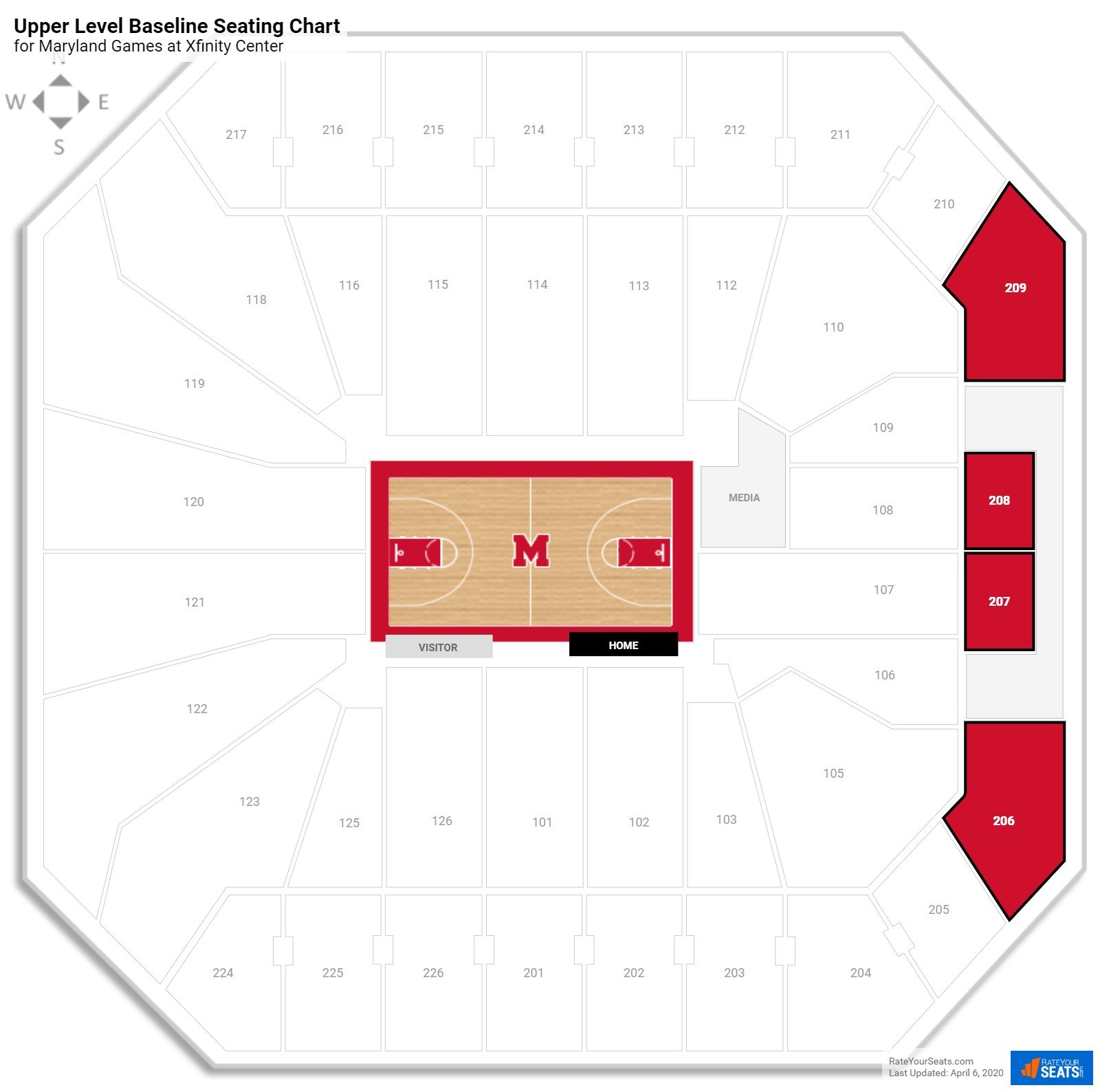This image displays the Upper Level Baseline seating chart for Maryland games at the Xfinity Center. Central to the chart is the basketball court, bordered in red, featuring red keys and a prominent red "M" representing the University of Maryland logo at center court. Highlighted on the far right side of the stadium are four red sections: 209, 208, 207, and 206, indicating the highest seats on the upper level's right side.

Adjacent to the basketball court's right edge is the media section. The seating sections closest to the court begin at 101, positioned at the center and encircling the court up to section 126. The upper-level seating extends from section 201, located directly behind section 101, and continues around the stadium to section 226.